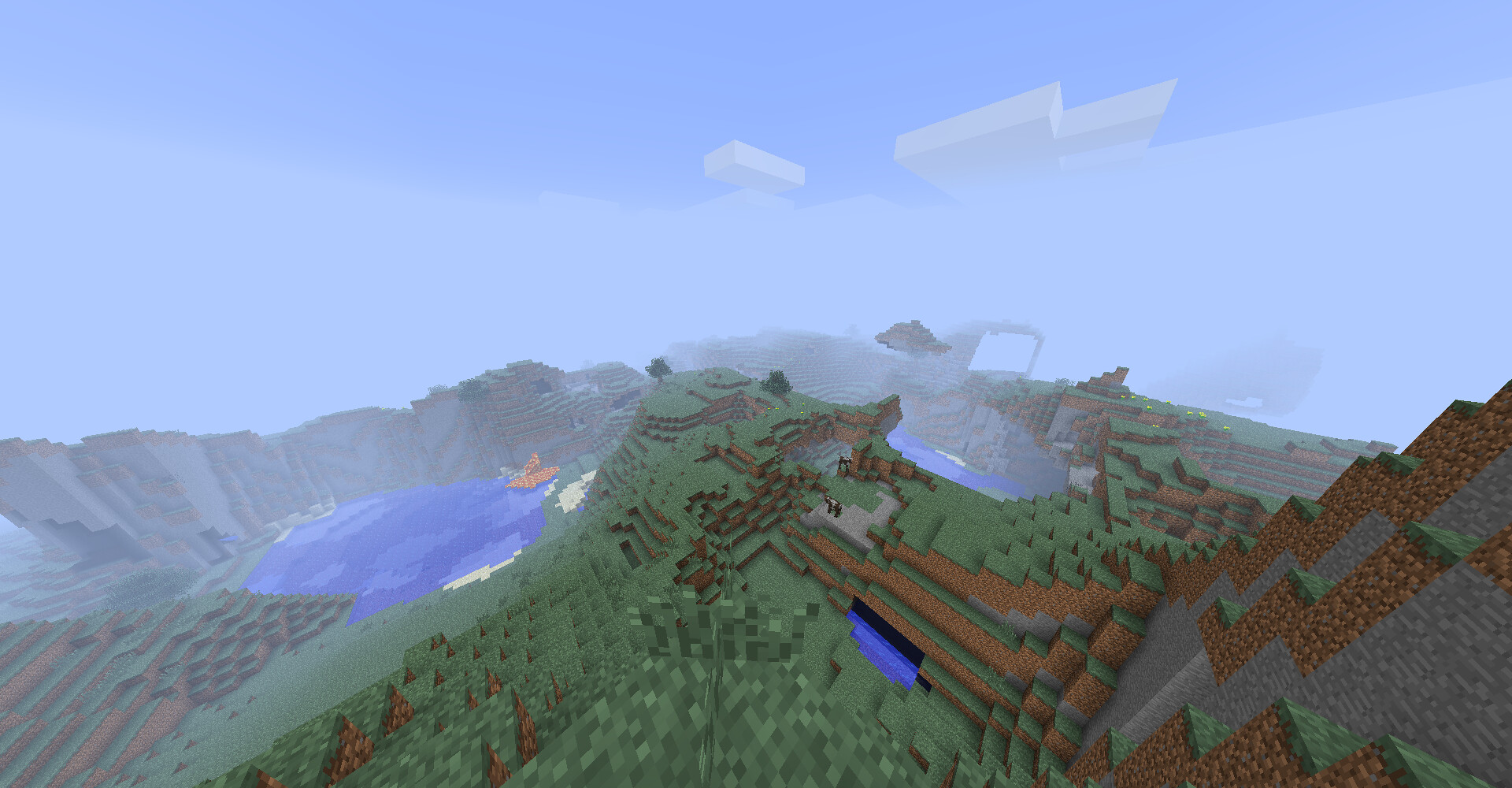This image presents a pixelated, aerial view of a landscape that resembles a grassy canyon, imparting a video game-like aesthetic with its blocky appearance. In the foreground, at the center lower part of the image, there is a prominent grassy hill. Towards the left, the landscape transitions into a deeper canyon resembling a quarry, characterized by its grayish tones. At the bottom of this canyon lies a round body of water. On the right-center portion of the image, another distinct canyon is visible, which also contains a small body of water. The pixelation and blocky features enhance the scene's resemblance to a digital or video game environment.